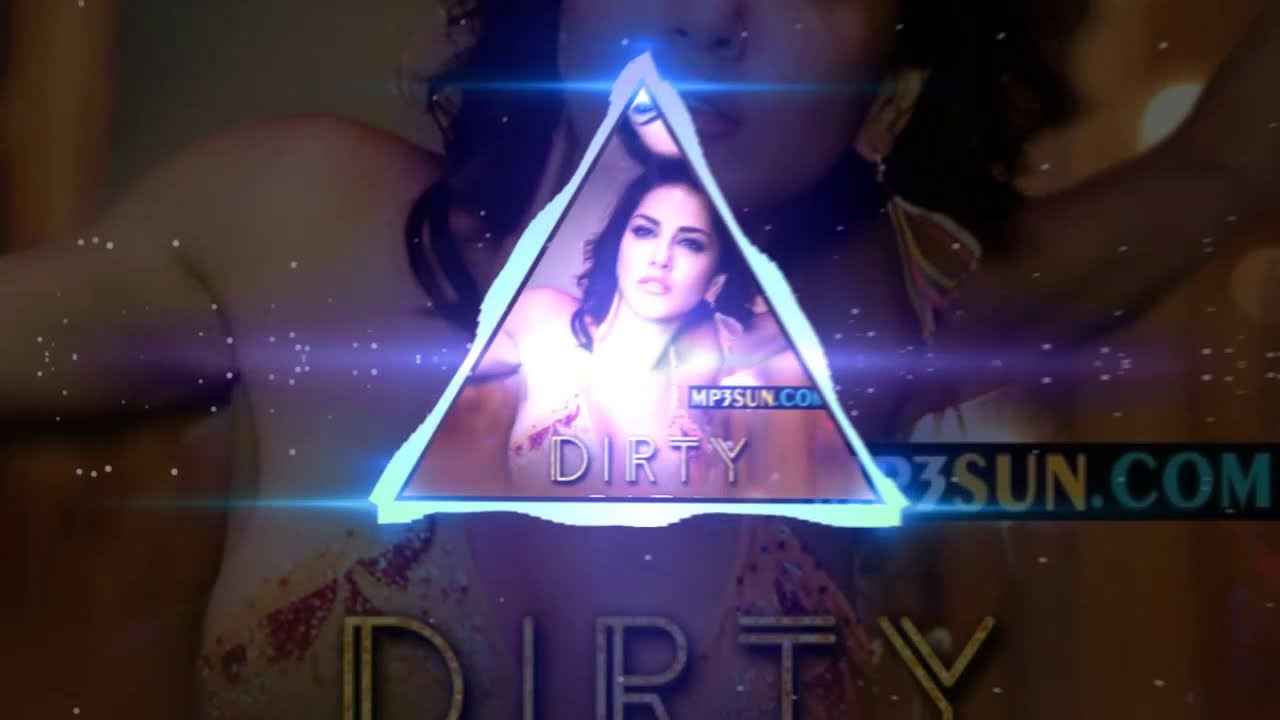This image appears to be a digital poster or song cover featuring a striking and detailed design. At the center is a glowing triangle with rugged edges, reminiscent of the Zelda logo, emitting sparkling rays from the left and right. Inside this triangle, there is a close-up of a woman with shoulder-length, dark hair. She is wearing a string bikini and exudes a sultry look, gazing just above the camera beyond the viewer. Superimposed across her chest is the word “Dirty” in double-lined text, and just above to the right of that, it says “mp3sun.com.” The background of the poster showcases a larger, zoomed-in, and shaded version of the same image, adding a layered depth to the overall design.